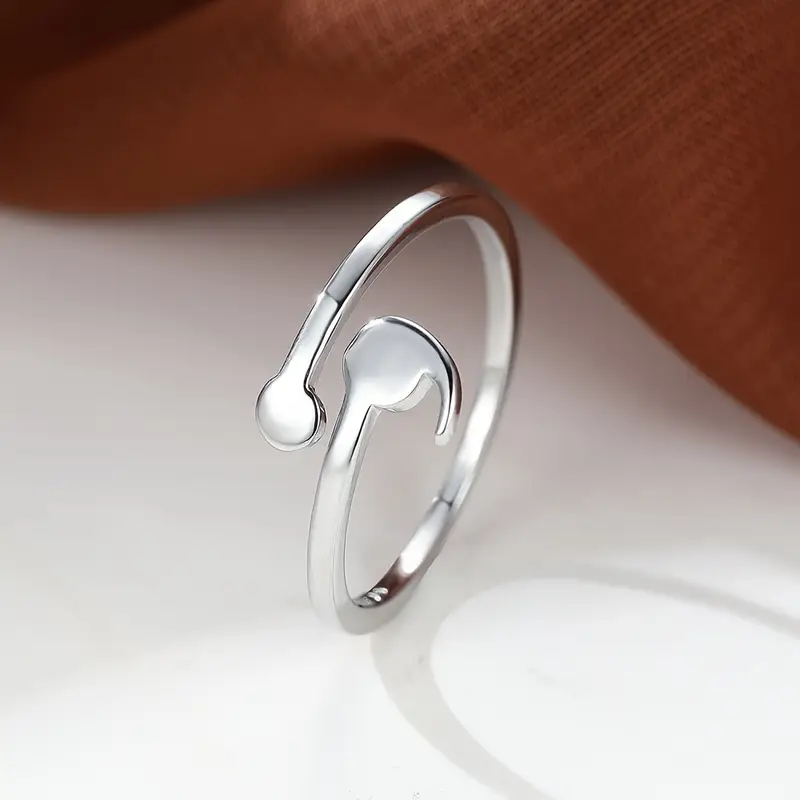This photo features a sterling silver ring displayed against a white background. The ring is not a continuous band; instead, its two ends overlap without touching, resembling an open bangle that has been formed into a circular shape but left not fully enclosed. One end of the ring is rounded like a ball, while the other end extends into a long, narrow part with a slight hook, giving the illusion of a tail. The metal is sleek and shiny, with visible engraving on the inside, though the details of the inscription are not clearly discernible. A light gray shadow is cast below the ring, adding depth to the image. Behind the ring, a skin-colored object, possibly a finger or a leg, peeks through, covered in a cross-hatched shadow pattern. Additionally, a rust-colored blanket, towel, or sweater is arranged in the background, contributing a touch of warmth to the otherwise minimalist composition.